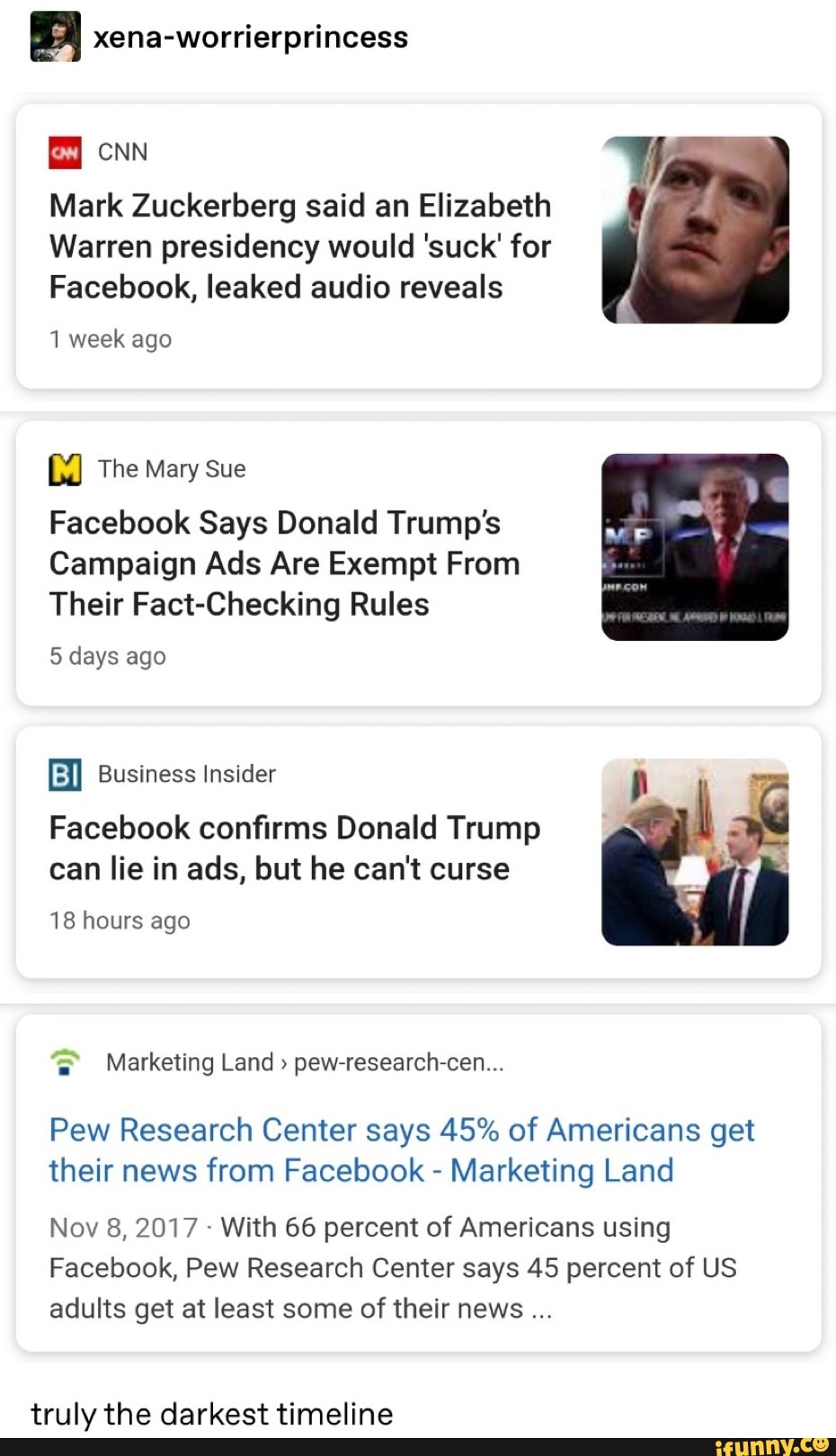**Screenshot of a News App on a Smartphone**

In the upper left corner, the screen displays the title "Xena: Warrior Princess." The first headline in the uppermost rectangle is from CNN, reading "Mark Zuckerberg said an Elizabeth Warren presidency would suck for Facebook, leaked audio reveals," accompanied by a picture of Mark Zuckerberg on the far right.

Below it, an article from The Mary Sue headlines "Facebook says Donald Trump's campaign ads are exempt from their fact-checking rules," featuring an image of Donald Trump.

Further down, a Business Insider article states "Facebook confirms Donald Trump can lie in ads, but he can't curse," with a small square photo showing Donald Trump shaking hands with, presumably, Mark Zuckerberg. This article was posted 18 hours ago.

The bottom rectangle contains a headline from Marketing Land referencing a Pew Research Center study: "Pew Research Center says 45% of Americans get their news from Facebook," dated November 8, 2017. The text notes that with 66% of Americans using Facebook, 45% of U.S. adults get at least some of their news from the platform.